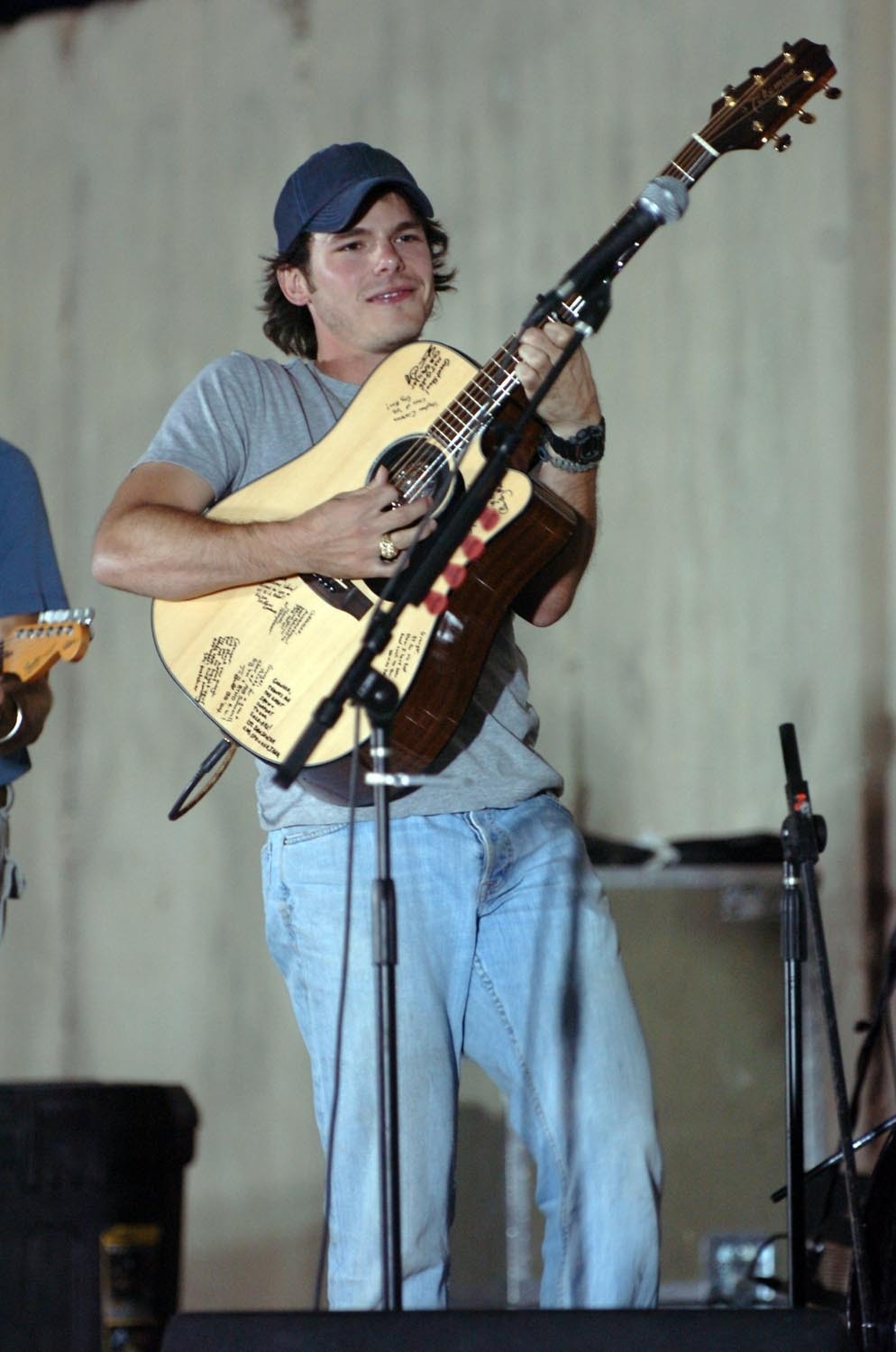In this outdoor photograph, we see a young man, possibly in his late teens or early twenties, passionately strumming a light wooden guitar, which features some indistinct writing or symbols on it. He is slightly smiling and gazing off to the right. He is wearing a blue baseball cap over his short to medium-length hair, a gray t-shirt, and well-worn blue jeans. His right arm is wrapped around the guitar while his left hand is positioned on the fretboard. In front of him is a microphone on a stand, indicating that he is in the middle of a performance. Despite the somewhat muted color palette of the scene, consisting mostly of grays and blues, the image captures a vibrant moment of musical expression. There is another person in the background to the left, only partially visible with just their head and instrument sticking out, further suggesting that the young man is part of a band. The background features a gray wall, and various pieces of equipment can be seen around the edges of the photo, hinting at a casual, live performance setting.